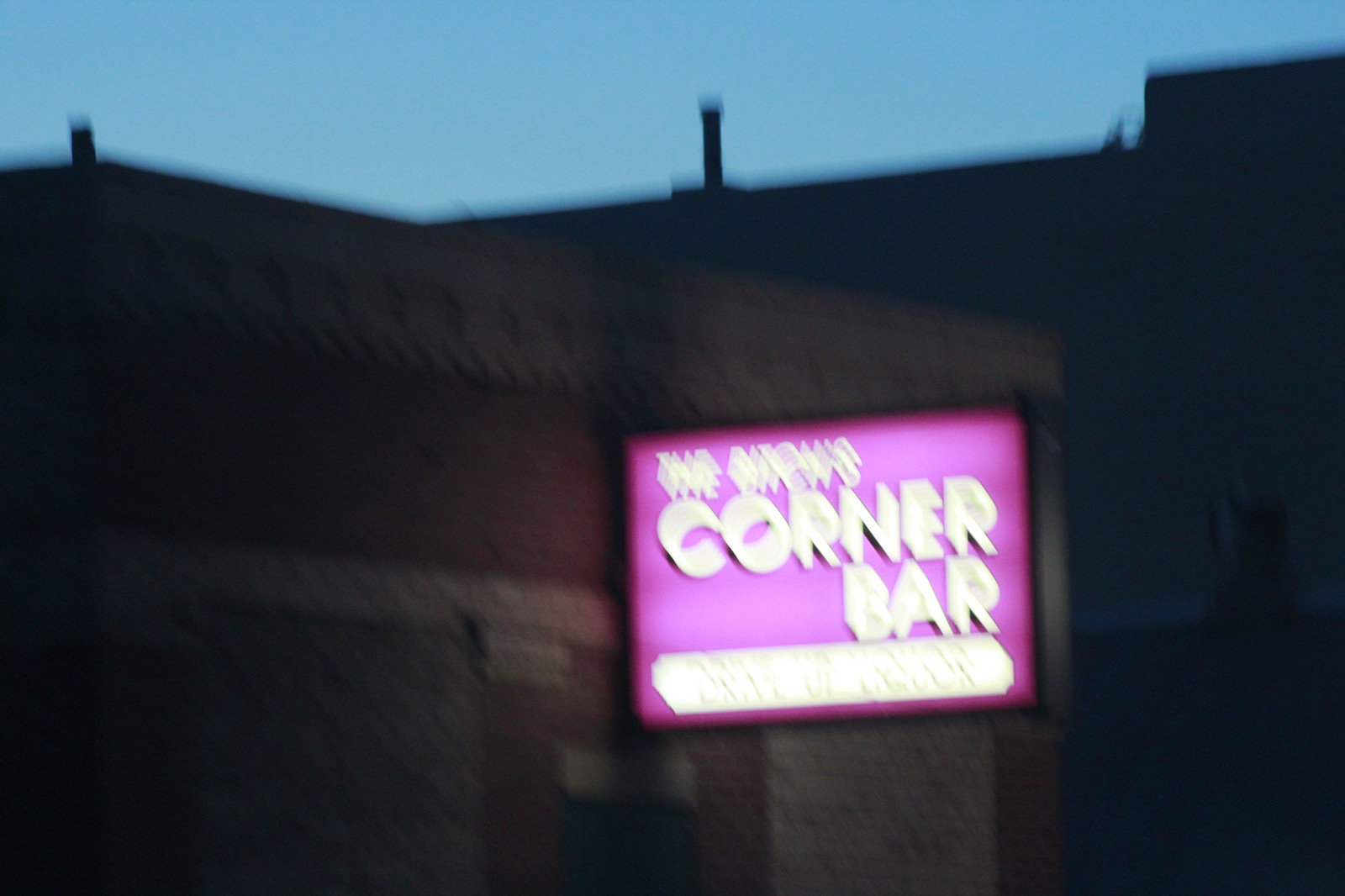The image is a blurry, out-of-focus photograph taken at dusk, showing a purple or pink LCD sign with a black frame that has white text reading "The Bitch's Corner Bar." The word "corner bar" is in larger text at the bottom, while "the bitch's" appears smaller at the top. The sign has indistinct and possibly yellow lettering beneath the “corner bar” text. Behind the sign is a small brick building in brown and tan tones, with a chimney extending above the roof. The sky in the background is a dimming blue, suggesting the photo was taken in the late afternoon or early evening. The setting appears outdoors, adding to the overall scene that includes multiple building structures.